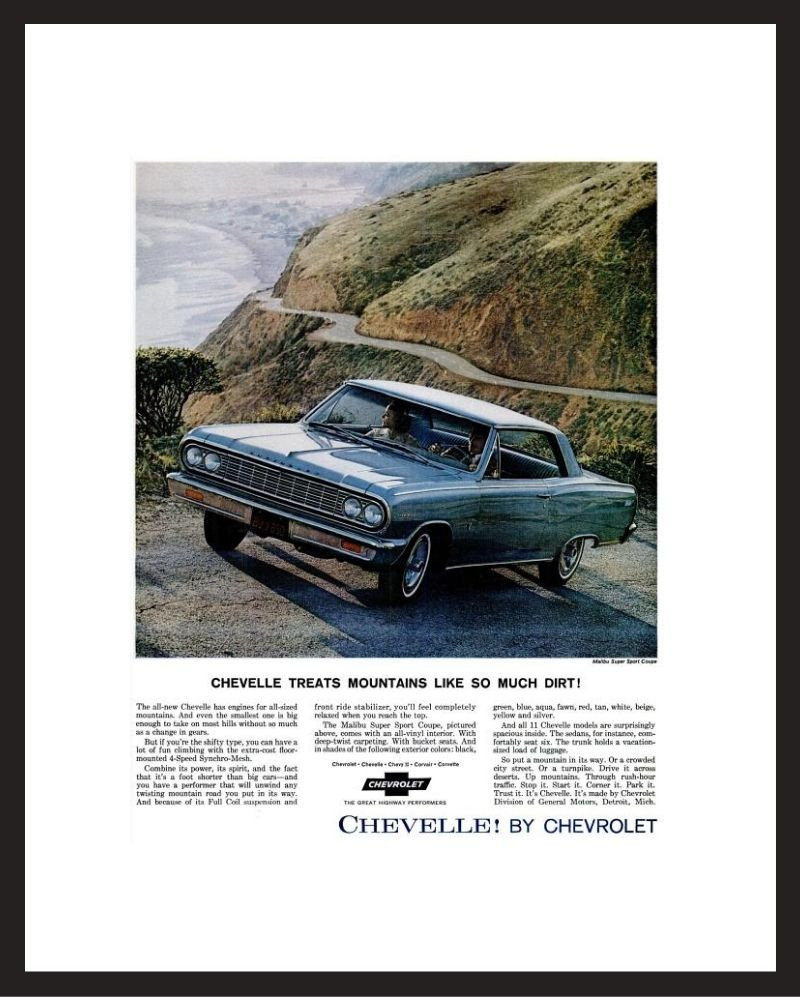The image is a detailed magazine advertisement for Chevrolet featuring a framed, picturesque scene centered around a blue Chevrolet Chevelle with a white top. Positioned prominently in the middle, the Chevelle navigates a winding mountain road that curves both above and below it, amidst lush green and yellow vegetation. To the left, the scene extends to a coastal view with the ocean and surf visible, completing the backdrop. The caption beneath the image reads, "Chevelle treats mountains like so much dirt," emphasizing the car's capability to effortlessly handle rugged terrain. Additional text elaborates on the Chevelle's performance, and the iconic Chevrolet logo is displayed below the detailed information about the car, reinforcing the brand identity.